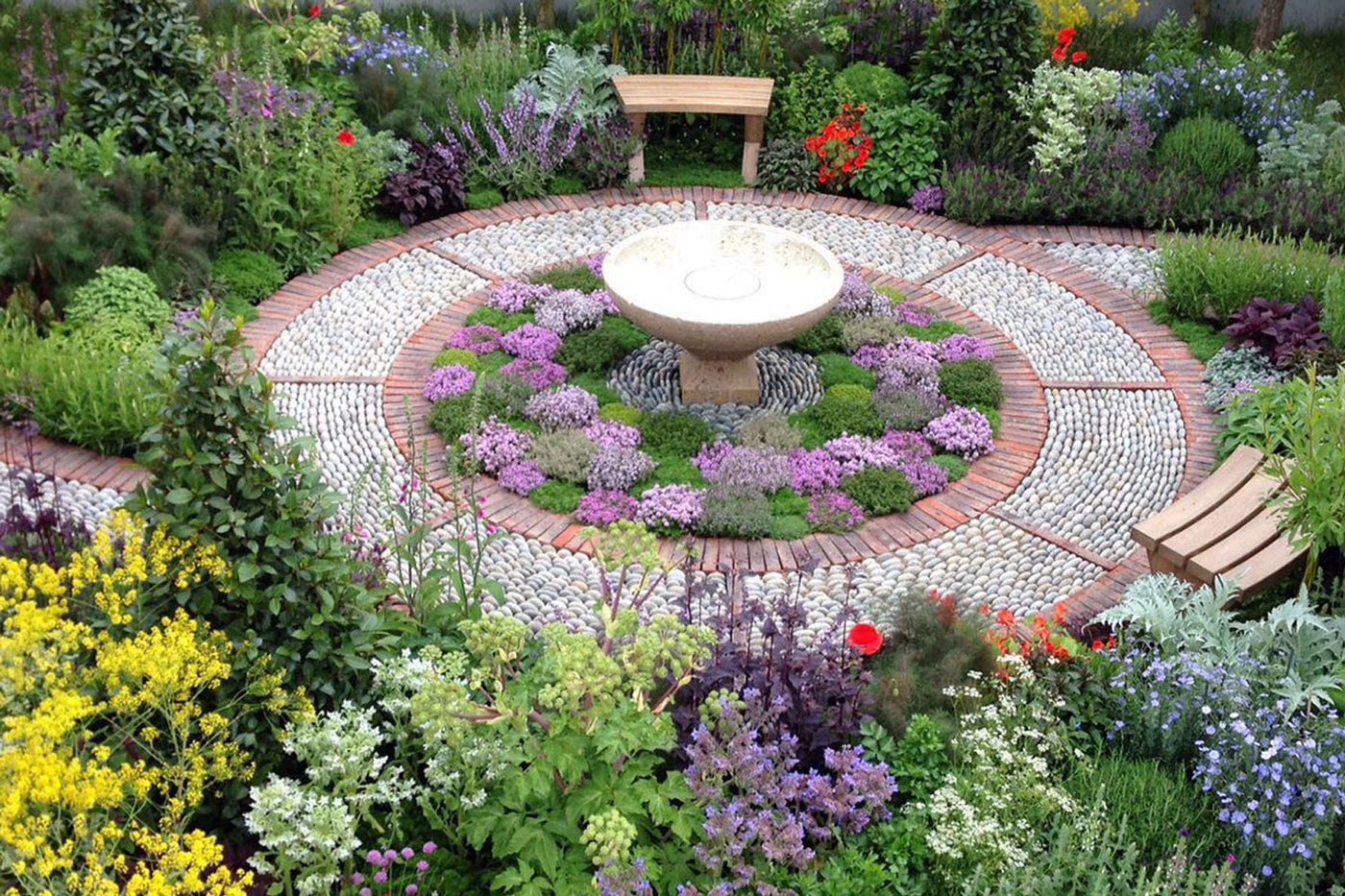In the center of a lush garden, a meticulously crafted circular stone arrangement stands out. The grey stone circle is accentuated by an inner and outer ring of red, with red lines radiating from the center, dividing the grey stones into segments. Encircling this stone feature is a vibrant array of green bushes adorned with flowers in a multitude of colors - purple, red, white, and yellow. Among the greenery, two well-placed wooden benches offer a place to sit and enjoy the surroundings. Dominating the central area of the stone circle is a striking white fountain, designed like a large bowl perched atop a pedestal, surrounded by a bed of purple flowers. Additional tree-shaped plants and blue flowers add to the garden's rich tapestry of colors. Pathways of stone extend to the left and top right of the visual, inviting further exploration of the serene and colorful garden space.